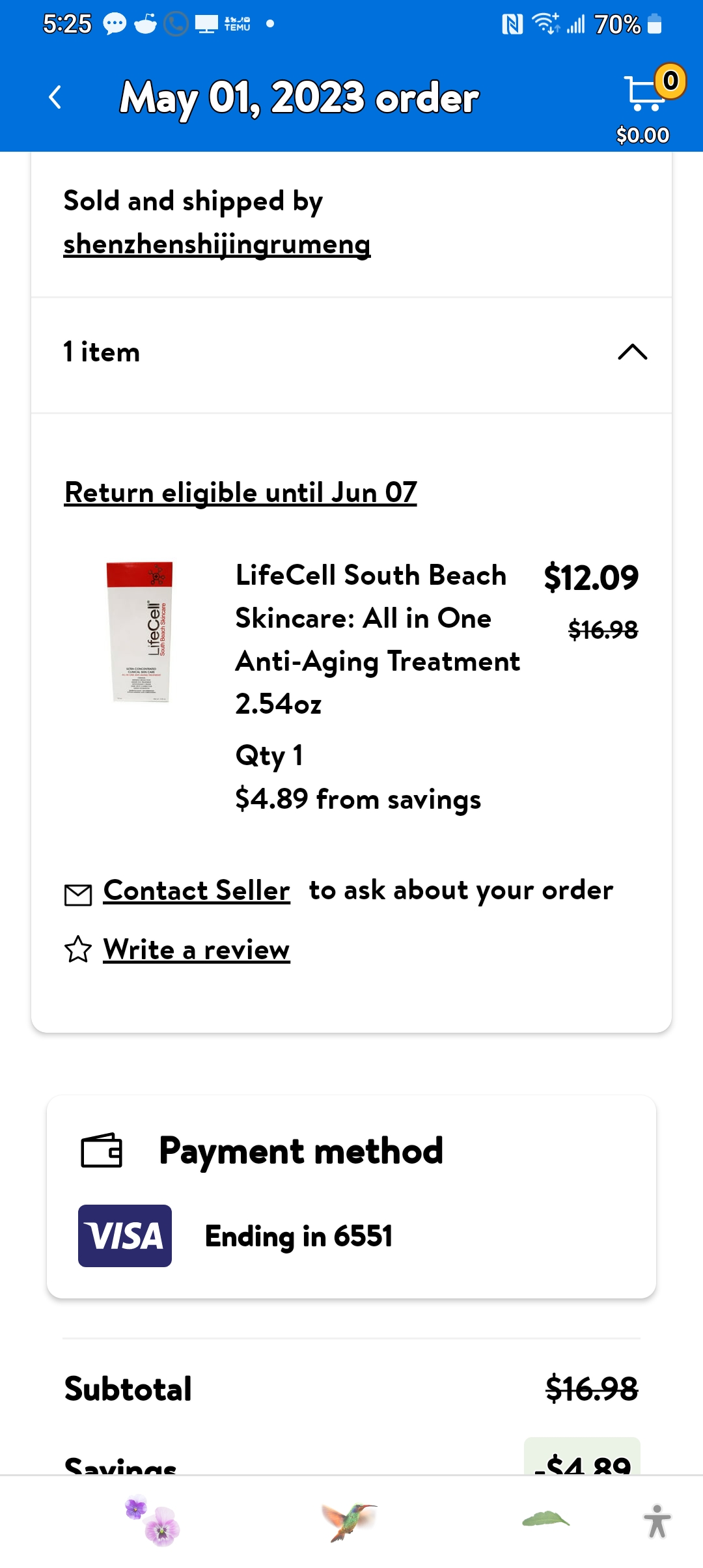The image is a vertically rectangular screenshot taken from a cell phone. At the top of the frame, a blue horizontal banner displays various interface elements. In the upper left corner, the time is shown as 5:25, and a series of icons indicate a 70% battery life, among other statuses. Positioned within the blue banner is a prominently bolded text stating "May 1st, 2023 order," accompanied by a shopping cart icon with a zero next to it, suggesting an empty cart. The overall design and font style hint at this being a Walmart interface.

The rest of the background is white, detailing the specifics of an order. It mentions "Sold and shipped by SHENCHENSHIJINGRUMENG," and notes that the return is eligible until June 7th. An image of the product appears on the left side, while to the right, the product's name and details are listed: "Life Cell South Beach Skin Care, All-in-One Anti-Aging Treatment, 2.54 ounces," with a quantity of one. The item's price is originally $12.09, but savings of $4.89 are applied, reducing the cost. Below this information, there are links to "Contact seller" and "Write a review."

Further down, the payment method is indicated by a Visa logo with the card ending in 6551. The subtotal is shown as $16.98 with a line through it, and only the top portion of the next line is visible, enough to read "savings" and the amount "-$4.89."